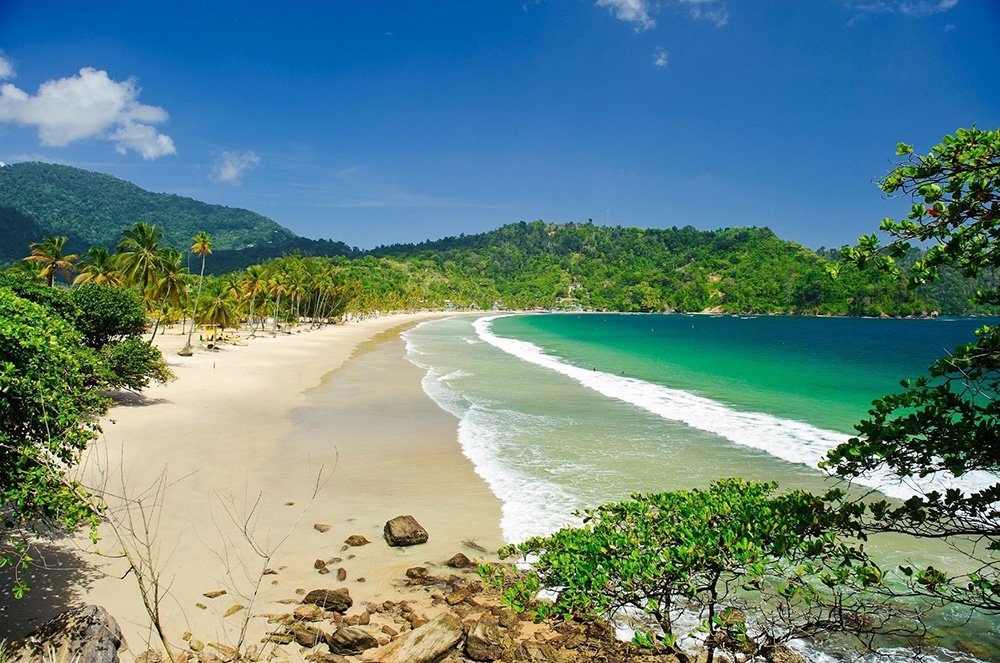The image captures a vibrant tropical landscape centered around a serene beach setting. Dominating the left side is a lush green mountain topped with a striking blue sky and a fluffy white cloud. The mountain slopes down into a densely forested area filled with towering pine and palm trees, giving a rich green backdrop. In the foreground, scattered pieces of wood and short green shrubs add texture to the scene, and thin tropical trees with characteristic palm fronds stretch upward.

Extending across the central part of the image is a prominent bridge, drawing a visual connection between the forested hillside on the left and the calm, inviting beach on the right. Adjacent to the bridge, the beach exhibits pristine white sand and gently breaking waves. The ocean's water near the shore is a serene green, transitioning to a darker green hue farther out into what appears to be a large bay. This bay, with its tranquil, turquoise tones, is encircled by the lush, rolling hills of the island.

Additional elements in the scene include several tourists, some of whom are wading in the calm waters, and a few scattered benches along the shore, enhancing the idyllic and peaceful nature of this small inlet. The sky overhead is clear, with just a few puffy white clouds, capturing the essence of a perfect tropical day.